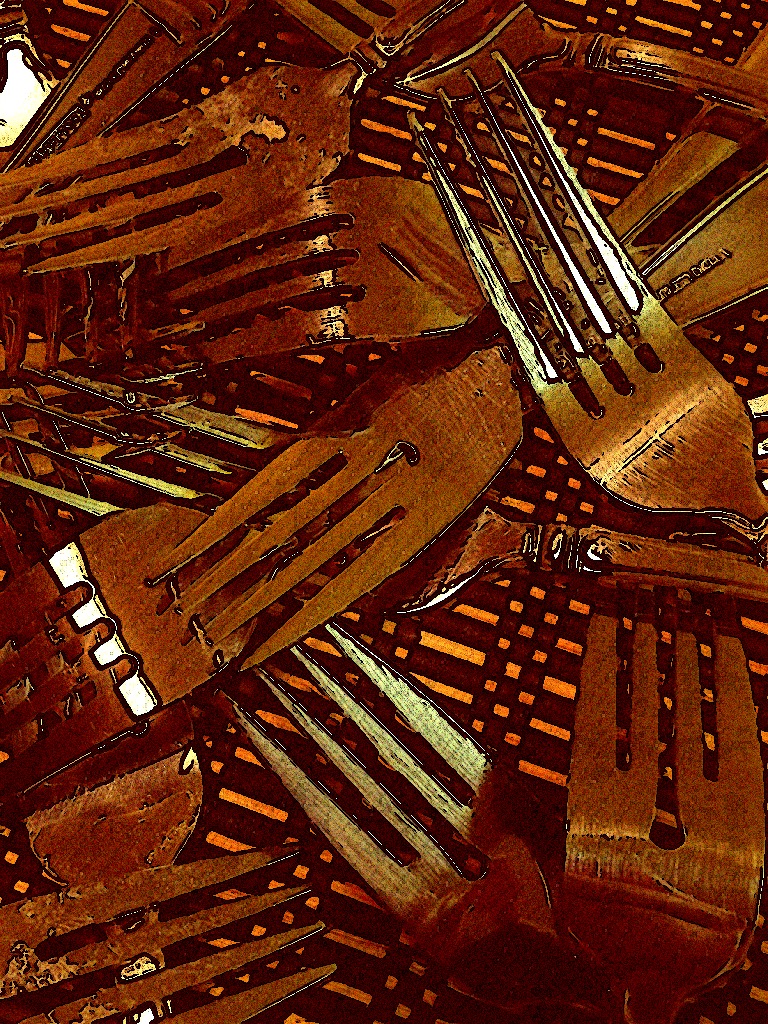This is a digitally altered, color-manipulated photograph of a collection of 10-12 silver dinner forks, all arranged with their heads visible and overlapping each other in varied directions. The image emphasizes an artistic flair, achieved through computer alteration to appear slightly overexposed, giving the scene a washed-out, nearly monochrome look. The details are slightly blurry, and some forks exhibit a subtle reddish-brown hue, possibly from the light reflection or digital editing. Despite the detailed arrangement, the background remains indistinct, focusing solely on the shiny, standard forks without any additional text or discernible setting. This visually striking image creates an impression of an artistic, graphic design composition rather than a straightforward photograph.